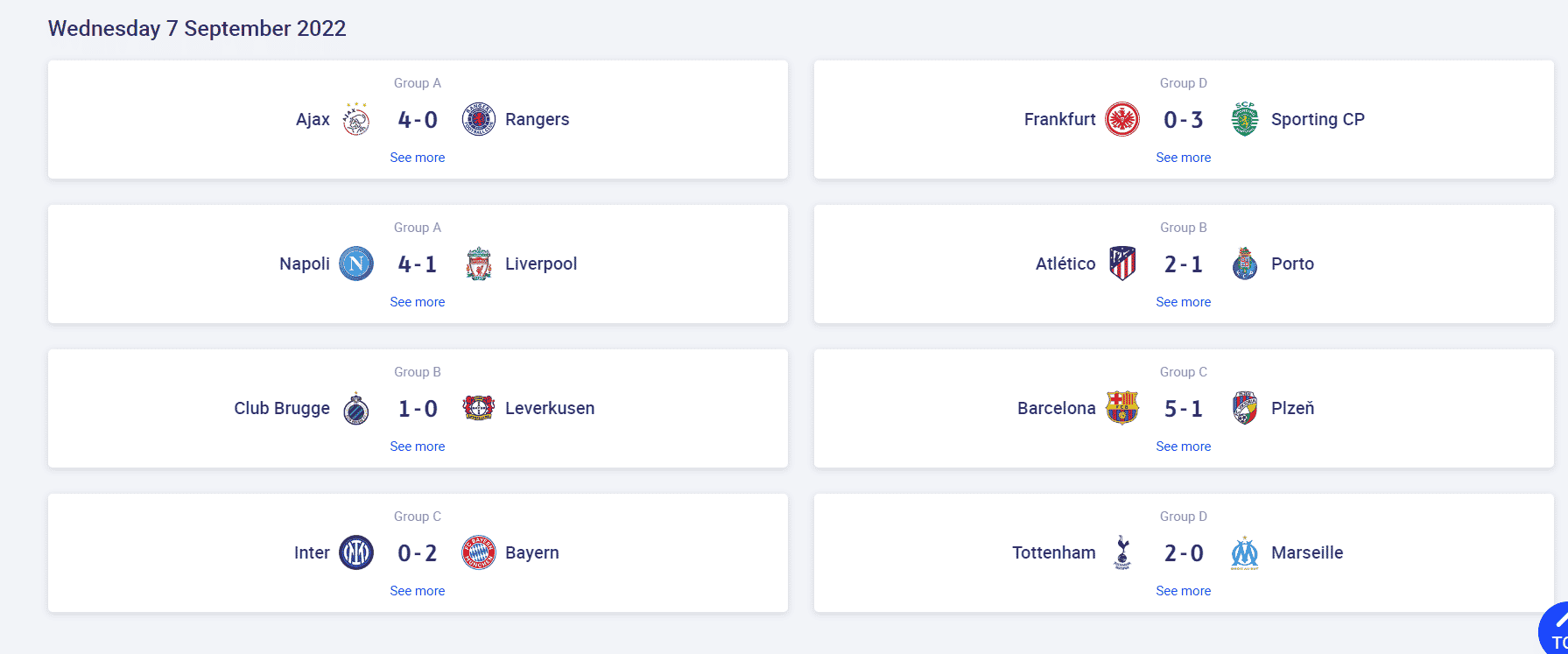The image displays a table of soccer (football) scores dated Wednesday, September 7, 2022, highlighted in a light purple-blue color at the top left corner. The table is organized into four rows and two columns, each entry presenting consistent information. At the top center of each score entry, the group designation is displayed, followed by the match details in the center, which include the home team, score, and away team. Beneath each entry, a "See More" link is shown in blue.

In Column 1:
1. Group A: Ajax (team logo) 4-0 Rangers
2. Group A: Napoli 4-1 Liverpool
3. Group B: Club Brugge 1-0 Leverkusen
4. Group C: Inter 0-2 Bayern

In Column 2:
1. Group D: Frankfurt 0-3 Sporting CP
2. Group D: Atletico 2-1 Porto
3. Group C: Barcelona 5-1 Viktoria Plzeň
4. Group D: Tottenham 2-0 Marseille

The table provides a clear and organized presentation of the match results, including team logos and precise final scores for each group stage game.